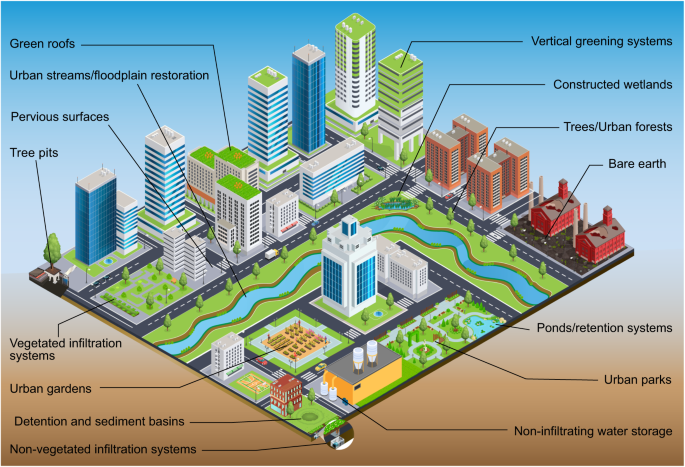This detailed image presents a complex, cartoon-like urban environment depicted as a 3D-infused, 2D street scene on a poster. The background transitions from a light blue gradient at the top to a darker brown gradient at the bottom. At the center of the image is a diamond-shaped city grid featuring an array of buildings, streets, rivers, trees, and parks. This city tile includes various elements such as skyscrapers with green and blue rooftops, apartment buildings, factories, and urban parks. A blue river snakes through the center, flanked by green areas with trees.

Surrounding the grid are numerous black arrows with labeled text pointing to different components of the scene. Notable labels include: green roofs, urban streams, floodplain restoration, pervious surfaces, tree pits, vegetative infiltration systems, urban gardens, detention and sediment basins, non-vegetative infiltration systems, non-infiltration water storage, urban parks, ponds retention system, bare earth, trees, urban forests, constructed wetlands, and vertical greening systems. Together, these elements appear to outline an environmental protection and urban planning strategy, emphasizing sustainable and green infrastructure development.